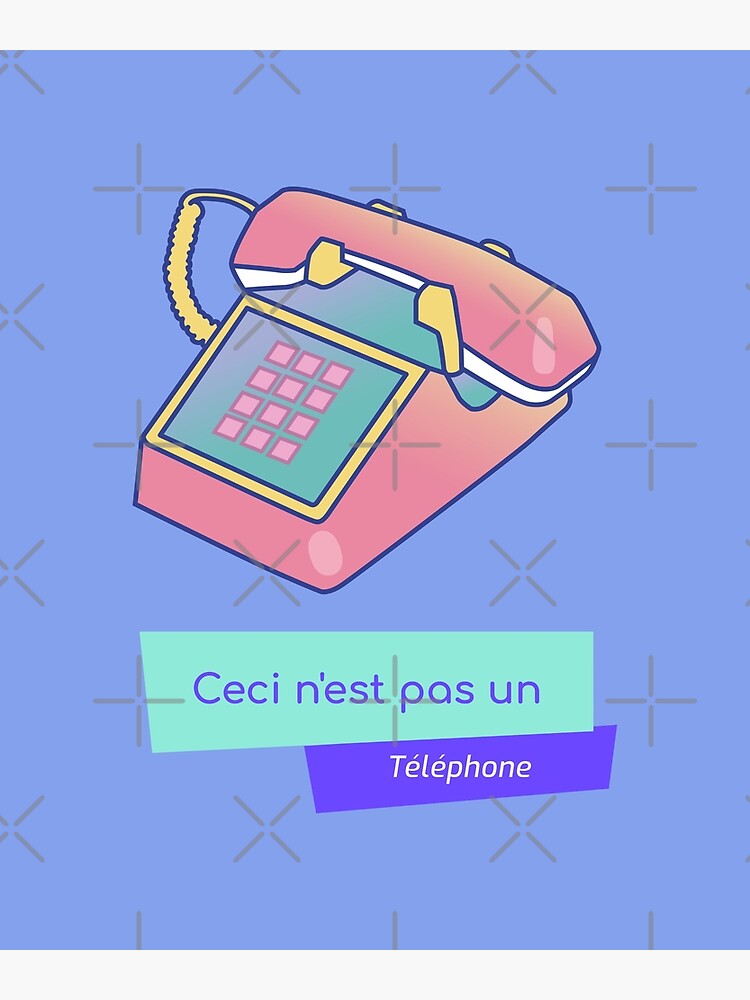The image is an advertisement featuring a cartoonish drawing of a vintage pink telephone, typical of the 1970s or 1980s. The phone has a pink body with a yellow cord and pink buttons where the numbers are dialed. It is set against a background of purplish-blue, which includes additional elements like stars, plus signs, and multiplication X’s scattered around. The phone rests on a green square panel with a yellow outline. Below the phone, there is a teal rectangular block with French text that reads "CECI N'EST PAS UN." Beneath this, there is a purple rectangle displaying the word "téléphoner" in yellow. The overall design evokes a retro aesthetic while incorporating playful geometric shapes and French phrasing.